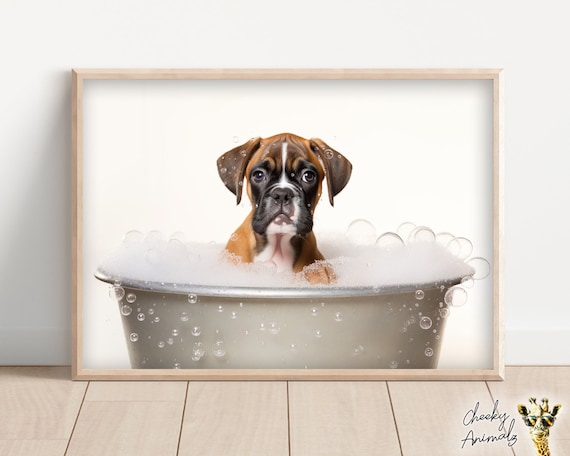This is an adorable, cartoon-style image of a bulldog in a bubble bath, framed in a thin, pale light brown frame. The bulldog, with floppy ears and brown, black, and white coloring, sits in a metal bath basin surrounded by a profusion of bubbles and suds. His expression is somewhat tired as he looks straight ahead, and his large brown eyes and a paw perched on the edge of the basin add to his charm. The setting is within a basic home interior with beige wooden floors and white walls, creating a simple, clean backdrop. In the bottom right corner of the image, the caption "Cheeky Animals" is displayed alongside a small drawing of a sunglasses-wearing giraffe, adding a playful touch to the scene.